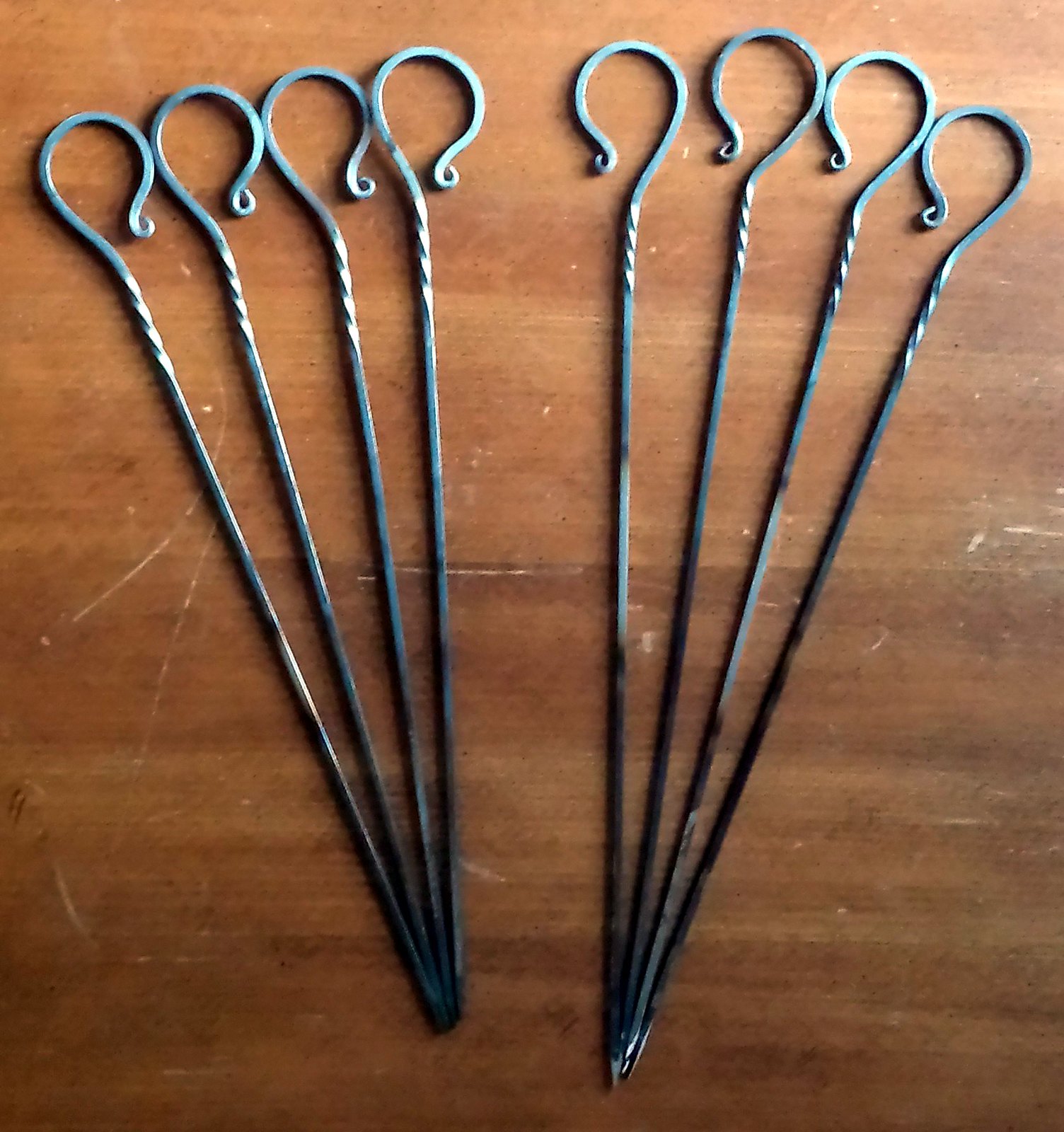This photograph captures eight wrought iron fire pokers meticulously arranged on a wooden surface. The pokers are divided into two groups of four, with a small gap separating them. Each poker is a long, silver metal piece culminating in a point at the bottom and fanning out towards the top. The top portion of each poker is intricately twisted, showcasing a spiraling pattern that leads to a large loop reminiscent of a shepherd's staff, complete with a tiny curlicue at the end. The pokers on the left side have their hooks facing right, while those on the right side are oriented left, creating a symmetrical arrangement where the pointed ends are close together, and the loops at the top also converge, forming a V shape or triangular outline. Notably, the lower halves of these pokers are blackened with soot, hinting at their use in fire, and they rest on a surface that appears to be either a well-worn wooden table or a scuffed wooden floor.